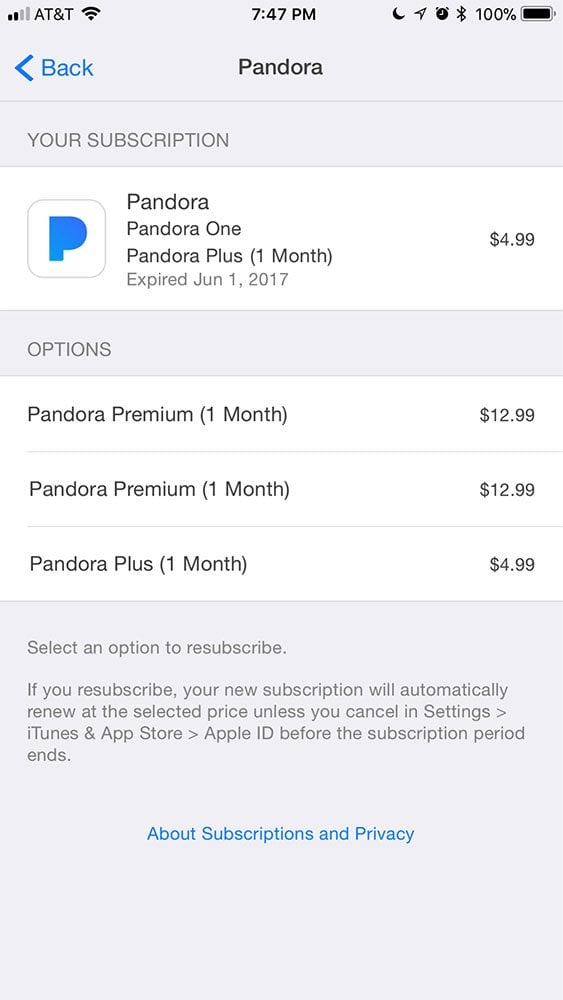The image is a screenshot from a smartphone with a very light gray background. In the upper right corner, the battery icon indicates a full charge at 100%. Adjacent to it, there are icons for Bluetooth and an alarm clock. The current time is displayed at 7:47 PM in the center top of the screen. The upper left corner shows the carrier name "AT&T" and a weak wireless signal indicator with only two out of five bars lit up, along with a Wi-Fi icon to its right.

Beneath the time, the app's header "Pandora" is visible. On the left side of this header, a blue "Back" button is accompanied by a left-pointing arrow. Underneath, a section with a white background displays subscription details. The prominently featured blue Pandora logo consists of a completely filled-in letter "P." Below the logo, text in gray font reads "Pandora," "Pandora 1," and "Pandora Plus," followed by "one month" and "expired June 1, 2017." To the right, the price "$4.99" is shown.

Further down, the options section offers three resubscription choices:
1. Pandora Premium (one month) for $12.99
2. Pandora Premium (one month) for $12.99 again
3. Pandora Plus (one month) for $4.99

The area below these options, against the gray background, prompts users to "select an option to resubscribe," with additional explanatory text. At the very bottom center of the screen, "about subscriptions and privacy" is displayed in blue font, likely indicating a hyperlink.